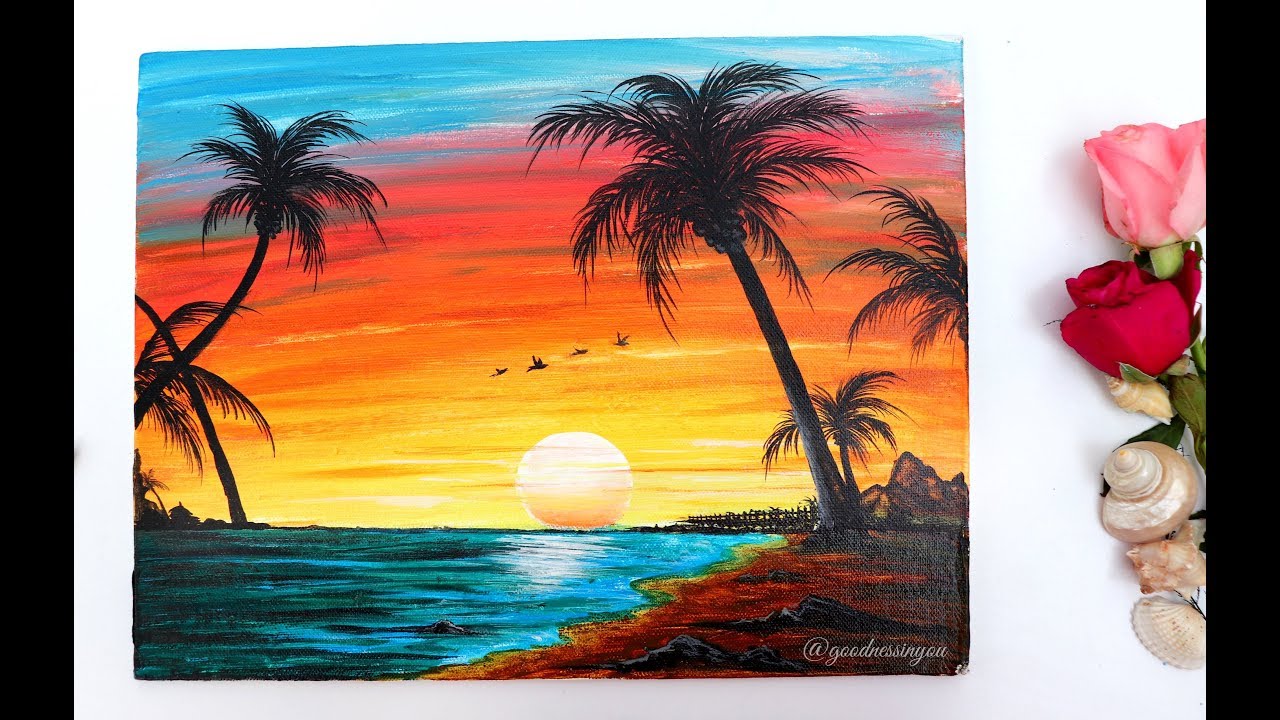This image showcases a painting mounted on a white background with thin black borders on the left and right. The vibrant painting centers on a tropical beach scene at sunset. The sky transitions from yellow near the horizon to deep orange, pink, and then blue as it rises, enhancing the four birds flying across. The setting sun appears to kiss the blue ocean on the left side, with tall palm trees standing gracefully on both shorelines. A small mountain range emerges on the right, complemented by sandy shores and rocks. Off to the right side of the painting, outside its frame, lies an artistic arrangement of a pink rose, a red rose, and three white, silver, and light pink seashells beneath them. The painting in a basic watercolor style exudes a serene ambiance, further accentuated by a handwritten tag reading "goodness in you" at the bottom right in lowercase cursive letters.